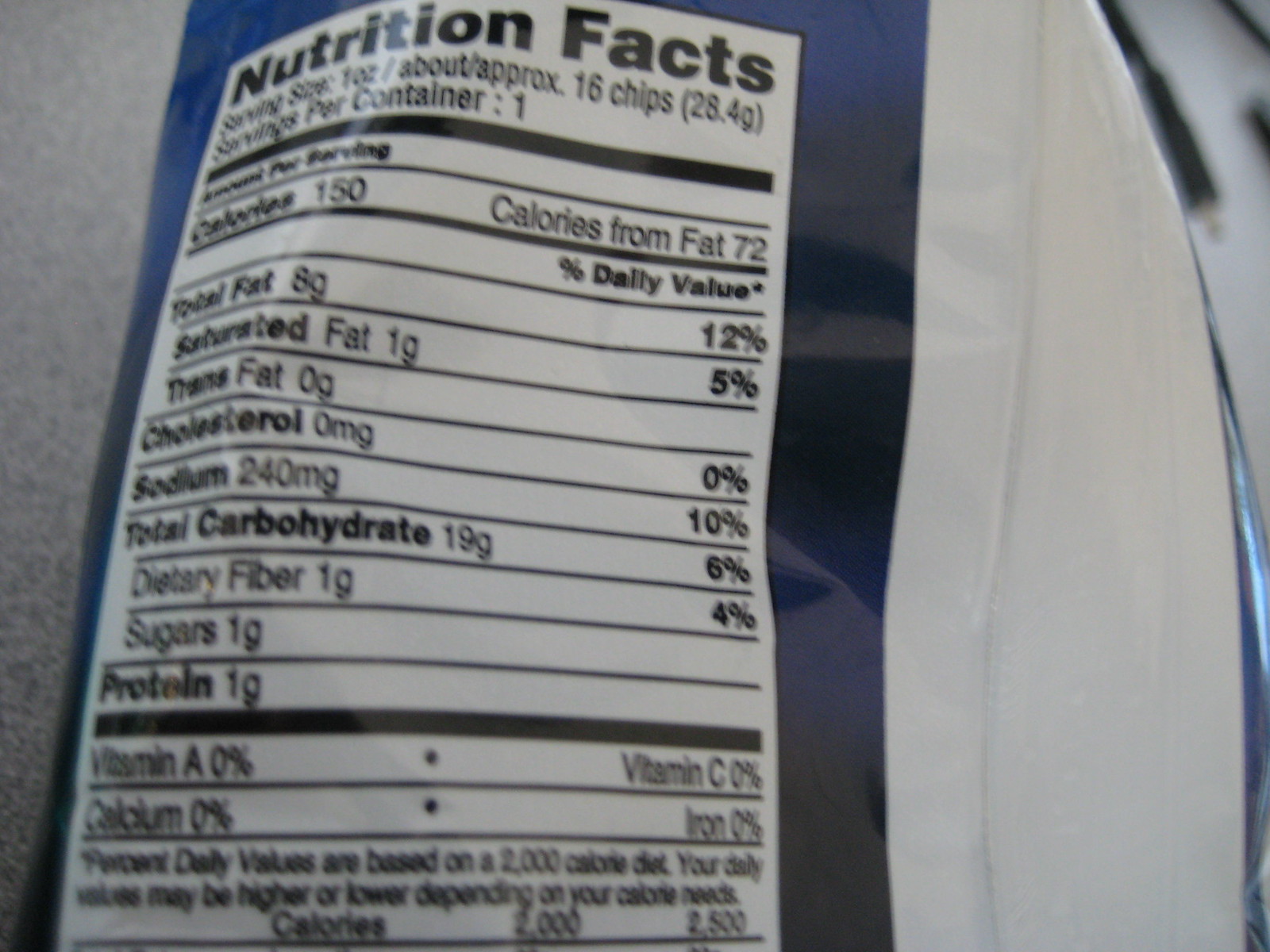The image captures a close-up of the nutrition facts table on the back of a blue bag of chips, adorned with white and light blue designs. The bag appears to be flexible and situated on a grayish background, with the nutrition table prominently displayed. The text, presented in bold black lettering against a white label, lists detailed nutritional information: serving size of 1 ounce (approximately 16 chips, or 28.4 grams), with a total of 150 calories. It includes 8 grams of total fat (12% daily value) with 1 gram of saturated fat (5% daily value) and 0 grams of trans fats. The cholesterol is at 0 milligrams (0% daily value), sodium at 240 milligrams (10% daily value), total carbohydrates at 19 grams (6% daily value) with 1 gram each of dietary fiber (4% daily value) and sugars. The protein content is 1 gram. Additionally, the vitamins and minerals section notes 0% for Vitamin A, Vitamin C, Calcium, and Iron. The table ends with a note stating that the percentage daily values are based on a 2,000 calorie diet.